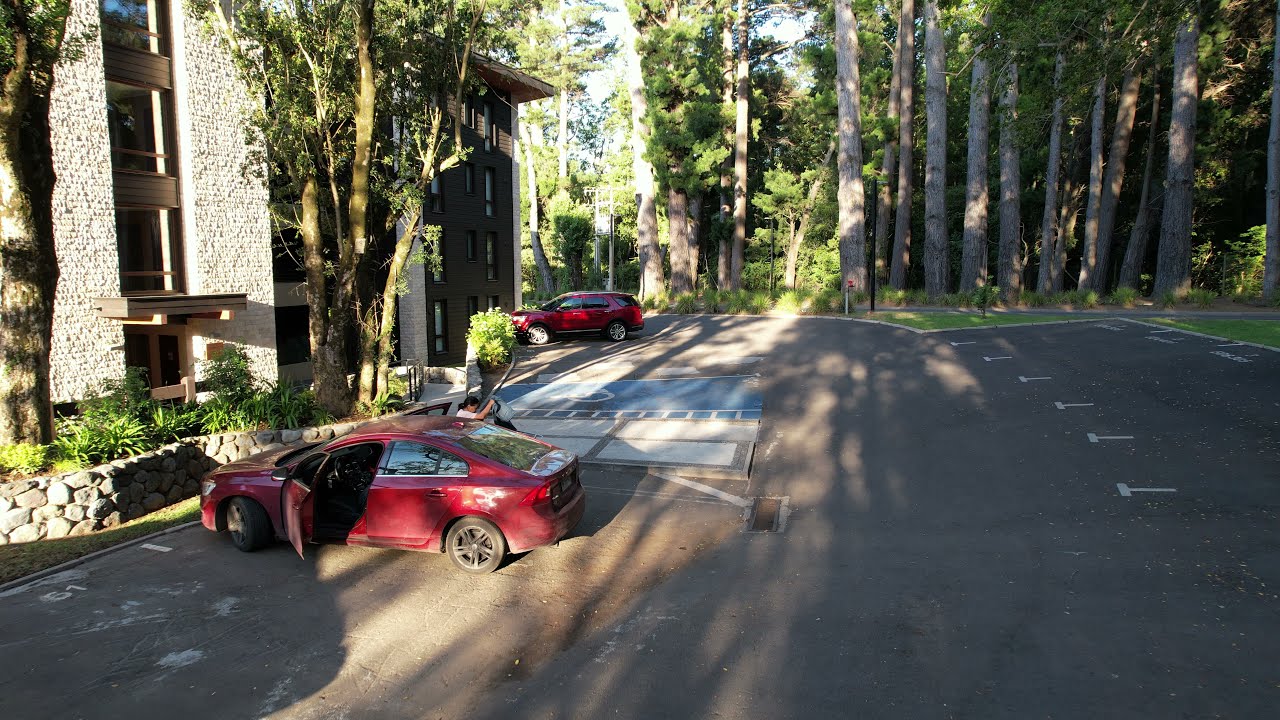The photograph captures a parking lot situated in front of a medium-rise building, likely an apartment complex or a hotel, characterized by its stone façade and wooden balcony accents. This building stands in a forested area, surrounded by towering trees with visible trunks and sparse leaves higher up, hinting at their immense height. The parking lot is largely vacant, demarcated with "T" shaped lines for parking spaces, and features a short stone wall that runs along part of its perimeter.

In the foreground, a red sedan with both the driver's and passenger side doors open is prominently positioned. A woman in a white t-shirt is by the passenger side, appearing to either don or remove a jacket. Further in the background, a red SUV is parked, similarly facing the building. The area exudes a sense of seclusion, underlined by the thick forest encircling it, suggesting it's possibly on the grounds of a resort or a remote residential complex.